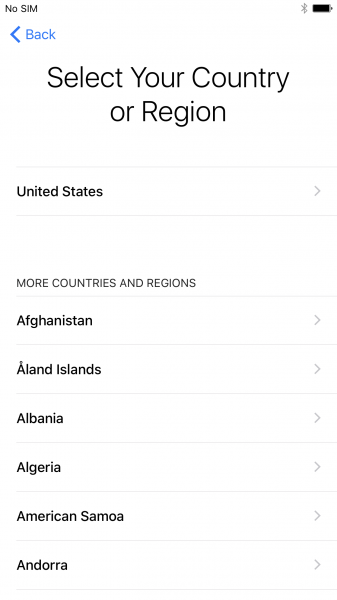The image depicts the initial setup screen of an iPhone running iOS, specifically the stage where the user is prompted to select their country or region. At the very top of the screen, a notification indicates that no SIM card is inserted into the device. The top right corner shows the Bluetooth icon, indicating that Bluetooth is enabled, and the battery icon, displaying a full charge of approximately 100%.

Below these indicators is a header text that reads "Select Your Country or Region," with "United States" pre-selected at the very top. To the right of this selection, there is a small arrow symbol hinting that tapping it will navigate to the next page. Below the United States option, a section labeled "More Countries and Regions" lists additional choices. These options are separated by thin gray lines and each has a small gray arrow pointing to the right.

Visible countries in this list include Afghanistan, Åland Islands, Albania, Algeria, American Samoa, and Andorra. The background of the screen is white, with all text in black, making the options easily readable. This screen represents one of the first steps in setting up a new iOS device, guiding the user through the necessary configuration process.